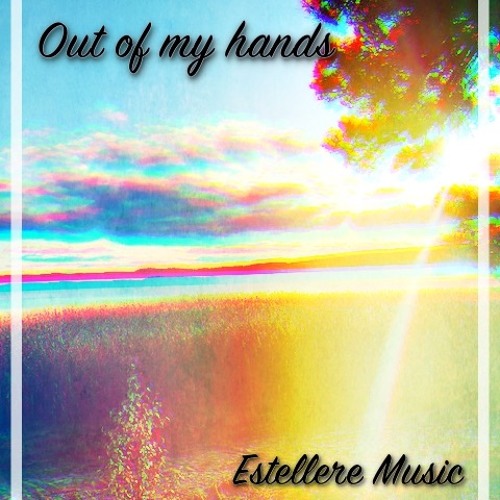The artwork is an album cover featuring a serene, slightly glitchy image that blends natural and painterly elements. The primary scene depicts a lakeside view with a distant hill or mountain, under a vibrant, colorful sky. A tree extends down from the top right corner, and sunlight filters through the clouds, casting a warm glow on the scene. The color palette includes prominent hues of blue, yellow, pink, and touches of red, creating a vibrant and slightly distorted effect.

At the top of the cover, the phrase “Out of My Hands” is inscribed in elegant black cursive with a shadow effect, mirroring the text at the bottom right corner which reads “Estellaire Music.” The words are framed by vertical white stripes on either side of the artwork. The design is highly detailed, colorful, and exudes a sense of tranquility despite its blurred and glitchy aesthetic. Overall, the cover blends natural beauty with artistic alteration, hinting at a musical journey by the artist Estellaire.